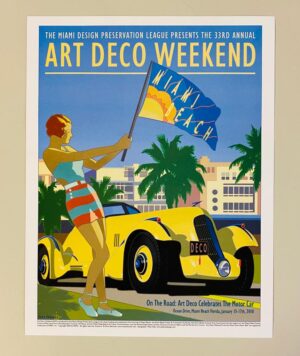The image is a small, rectangular vintage poster for the "33rd Annual Art Deco Weekend" presented by the Miami Design Preservation League. Framed with a light tan-brown and white border, it features an illustration of a woman with short reddish-brown hair, dressed in a blue halter top and a blue and red horizontal striped skirt. She sports white shoes and extends her arms to the right, holding a blue flag that reads "Miami Beach" with a small yellow-orange sun in the lower left corner.

In the background, against a blue sky, the title "Art Deco Weekend" is prominently displayed in large yellow, underlined lettering. Below the title, smaller text reads "The Miami Design Preservation League presents the 33rd Annual." The scene also includes a yellow 1950s-style sports car, palm trees, and a large white building resembling a resort or mansion. Although some text in the lower right-hand corner is too small to read, the overall composition captures a nostalgic and vibrant celebration of Art Deco influences in Miami Beach.